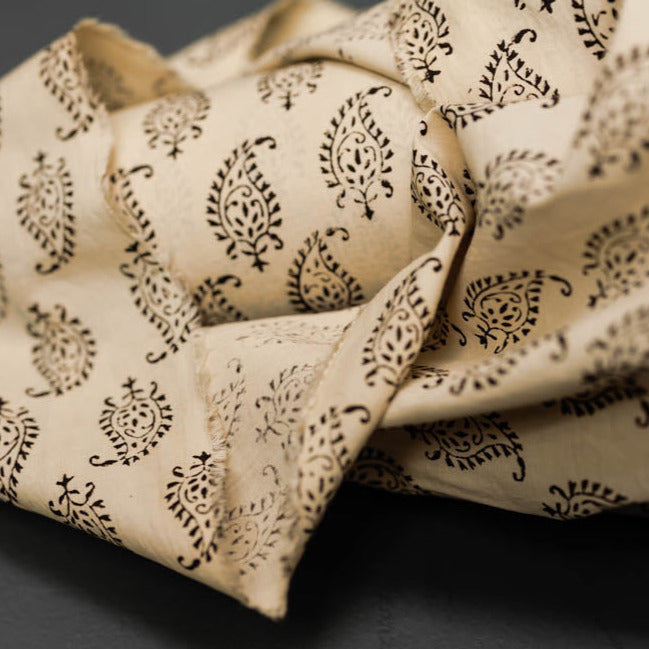The image depicts a close-up photograph of a white or cream-colored linen fabric sample, featuring a repeating black pattern that resembles a leaf or a many-legged, leaf-shaped insect. The design is printed all over the fabric, with some of the roll partially unrolled to reveal both the exterior pattern and a glimpse of the plain interior. The fabric is slightly crumpled and lays on a plain, dark background, possibly a black table or floor. The photo focuses on the fabric, with no other objects or people visible, and the texture appears suitable for furniture upholstery or drapery, rather than clothing.